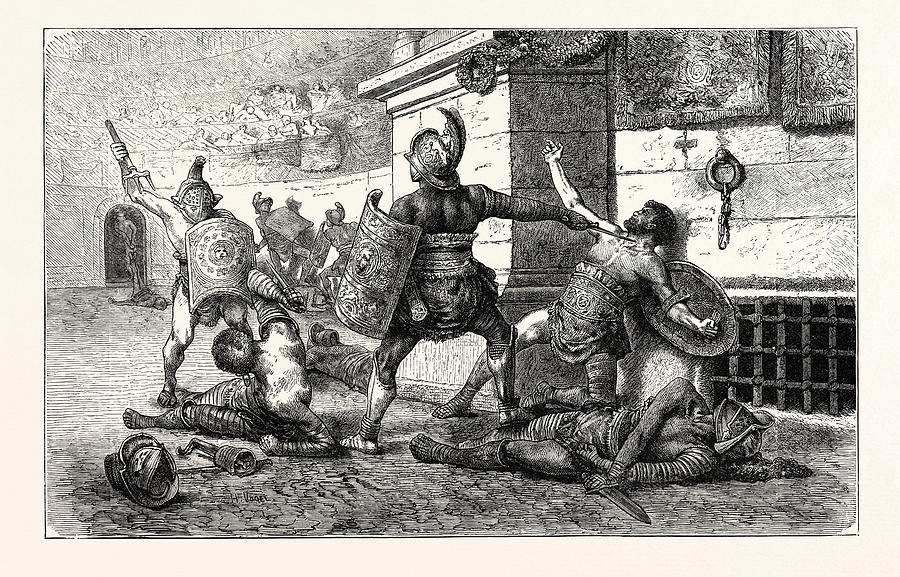This rectangular black-and-white illustration, set against an off-white, aged-paper background, is framed by a thin black line. The highly detailed, stippled and hatched drawing depicts a chaotic medieval combat scene inside a coliseum-like structure. Armored gladiators, equipped with shields, swords, and tridents, are engaged in brutal battles. Several figures lie injured or dead on the ground amidst a scattering of weapons and debris. In the scene’s foreground, one gladiator looms menacingly over another, sword poised at his neck, while another pair struggles, one raising his arm to fend off a trident attack. In the background, silhouetted figures continue to clash, while a sparse audience, depicted as simple circles and ovals, watches from multiple levels in the upper left corner. An arched doorway and a central column add architectural context to the setting, enhancing the overall atmosphere of ancient gladiatorial combat.